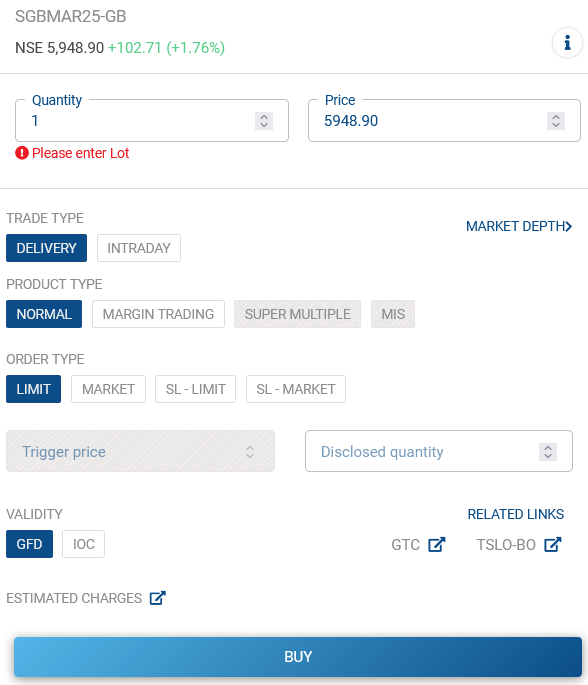The webpage details a real-time stock trading interface for purchasing shares on the stock market. The specific stock has a ticker symbol NSE and is currently priced at $5,948.90 per share, reflecting an increase of $102.71 or 1.76% today, highlighted in green. 

The interface has several sections:

- **Purchase Details:** Indicating a request to purchase one share. The label "Quantity" is in blue with the corresponding number (1) also in blue. The price $5,948.90 is similarly highlighted in blue. A red exclamation mark accompanied by a note "please enter lot" signals a requirement for additional input.
  
- **Trade Type:** Offers options like "Delivery" and "Intraday," with "Delivery" selected in blue. 
  
- **Product Type:** Choices include "Normal," "Margin Trading,” "Super Multiple," or "MIS." "Normal" is selected in blue, while "Super Multiple" and "MIS" are grayed out.
  
- **Order Type:** Available options are "Limit," "Market," "SL Limit," and "SL Market," with "Limit" selected in blue.
  
- **Trigger Price:** Features a gray text box with "Trigger Price" written in blue next to it.
  
- **Disclosed Quantity:** This is labeled in blue.
  
- **Validity:** You can choose between "GFD" or "IOC," with "GFD" selected in blue. 
  
- **Related Links:** This section includes clickable blue text for navigation to further information. Additional clickable options like "GTC," "TSLO," and "BO" are also presented.
  
- **Estimated Charges:** Mentioned with a link for further details that can open in a new window.
  
- **Purchase Option:** At the bottom, a prominently highlighted "Buy" button in white text on a dark blue background allows execution of the stock purchase.